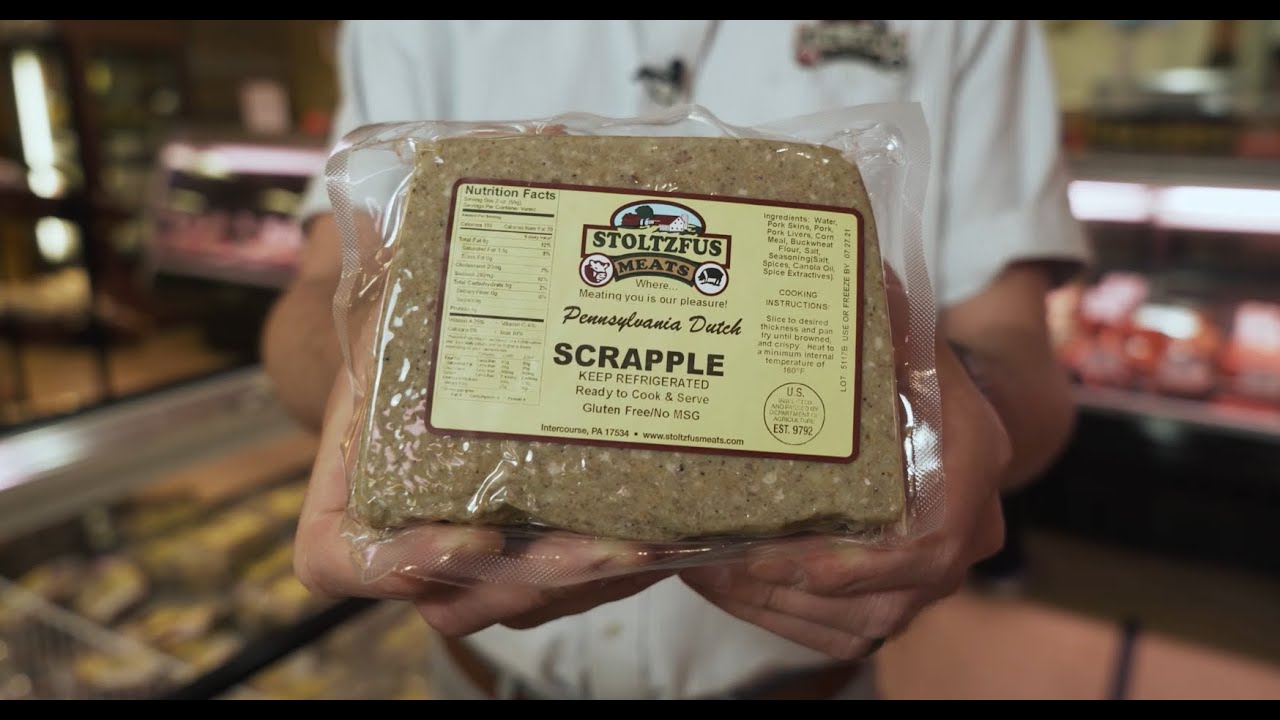This photograph captures a detailed moment in a butcher shop where a butcher, wearing a white short-sleeved shirt, is prominently holding a vacuum-sealed package of Pennsylvania Dutch Scrapple from Stoltzfus Meats. The man’s out-of-focus torso, visible from the chest down to his belt, occupies the center of the frame as he extends the package towards the camera with both hands. The label on the grayish-tan Scrapple, adorned with a farm logo and the text "Stoltzfus Meats," highlights that the product is ready to cook and serve, gluten-free, and free of MSG. Additional details such as nutrition facts and ingredients are present on the label. Behind the butcher, there are glass display counters containing an assortment of brown and orangish meat products, although they remain out-of-focus, along with a tan floor and indistinct tables or furniture suggesting a store or food production facility setting.